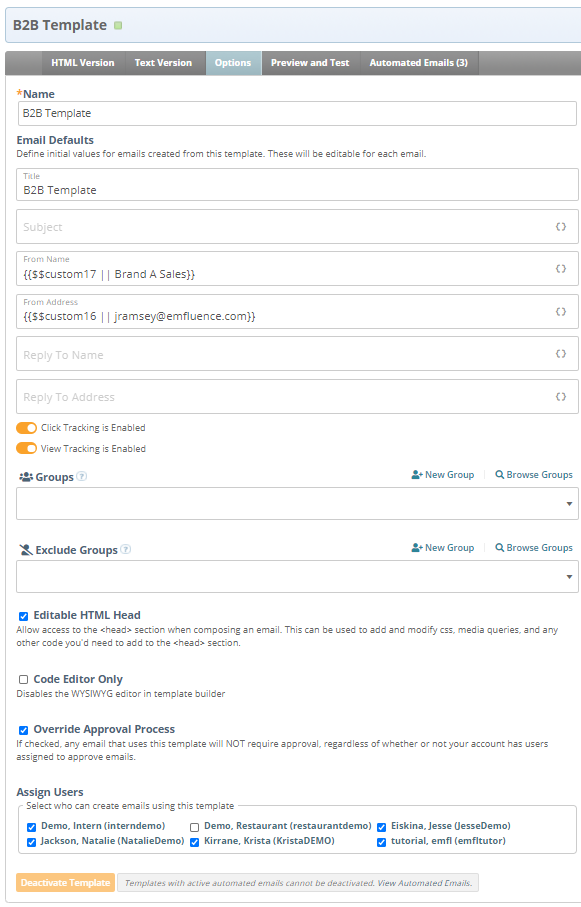This image showcases a clean, structured B2B (Business-to-Business) template on a web interface. The backdrop is predominantly white, occupying about 95% of the screen, framed by a subtle gray border. A light blue area spans horizontally across the top-left corner, where "B2B Template" is prominently displayed in bold, dark gray text. Adjacent to the text is a small green square.

Below this section is a slender, dark gray horizontal bar. Slightly to the right, but still aligned on the left, "HTML Version" is written in white, followed by "Text Version," also in white. To the right of these labels, a light blue segment marked with "Options" is visible, printed in white. Further right, "Preview" and "Test" appear, again in white. Just below lies a label "Automated Emails," separated by three hyphens, also in white.

The remainder of the page maintains a pure white backdrop, featuring distinct menu sections. The first menu on the left is highlighted by an orange star icon followed by the word "Name" in black text. Below this, a menu button states "B2B Template" in dark gray. Subsequent text "Email Defaults" is rendered in bold, dark gray, with a description beneath in lighter gray font: "Define initial values for emails created from this template. These will be editable for each email."

Continuing down, a horizontal, light gray-outlined rectangle holds "Title" in light gray, with "B2B Template" written inside in dark gray. Further below, another gray-outlined rectangle reads "Subject" in light gray, featuring a refresh button to the right. Descending further, yet another gray-outlined rectangle presents "From Name" in light gray at the top left, with "$$CUSTOM_17//Brand A Sales" written in dark gray.